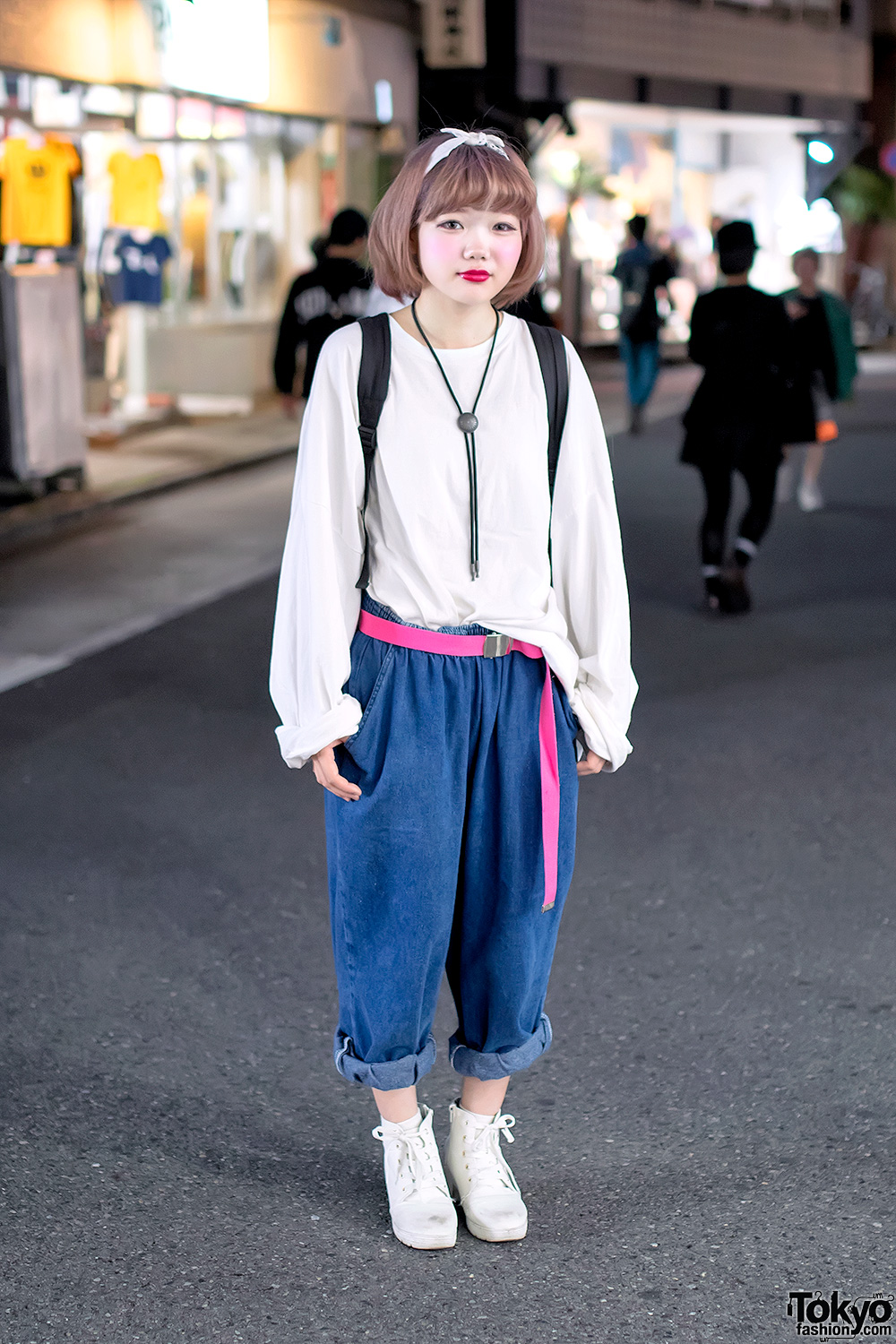In this vibrant street photo, a young Asian woman, possibly in her early twenties, stands prominently in the center of a bustling market street. She has a fair complexion and light brown hair styled above her shoulders with long bangs, adorned with a distinctive white bow. Her face is accented by bright red lipstick and faint makeup on her cheeks.

She is dressed in a loose, baggy white long-sleeve shirt, its cuffs rolled up, paired with equally baggy blue jeans that are rolled at the ankles, revealing her white high-top tennis shoes. Her outfit is accessorized by a striking pink belt with a long, dangling end and a black string necklace featuring a small circular pendant. She carries a black backpack slung over her shoulders.

To her left, blurred market stalls display various clothing items, hinting at shirts and other apparel. Background elements show several people milling about, some wearing black or green jackets, contributing to the lively street scene. The image is subtly marked with "tokyofashion.com" in the lower right corner, anchoring its urban and modern setting.